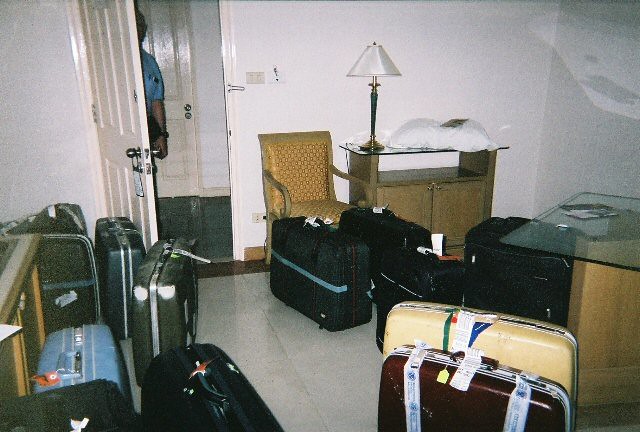The photograph captures an all-white room with pristine polished tile floors and white painted walls, giving it a bright and clean appearance. Centrally, the room is packed with various upright suitcases, predominantly black, each adorned with distinctive luggage tags—some of which are red. A noticeable yellow hard case and a burgundy hard case add splashes of color, along with a blue suitcase and a green one scattered among them. In the upper right corner, there's a small console table topped with a sleek, tall lamp featuring a white lampshade and a brass base. A tan armchair with golden upholstery sits to the left of the table. The table itself appears to have a piece of fabric or possibly a pillow resting on its glass surface. To the left of this setup, a partially open white door reveals a glimpse of someone standing just outside, dressed in a light blue short-sleeved shirt, hinting at a sense of surveillance or intrusion.